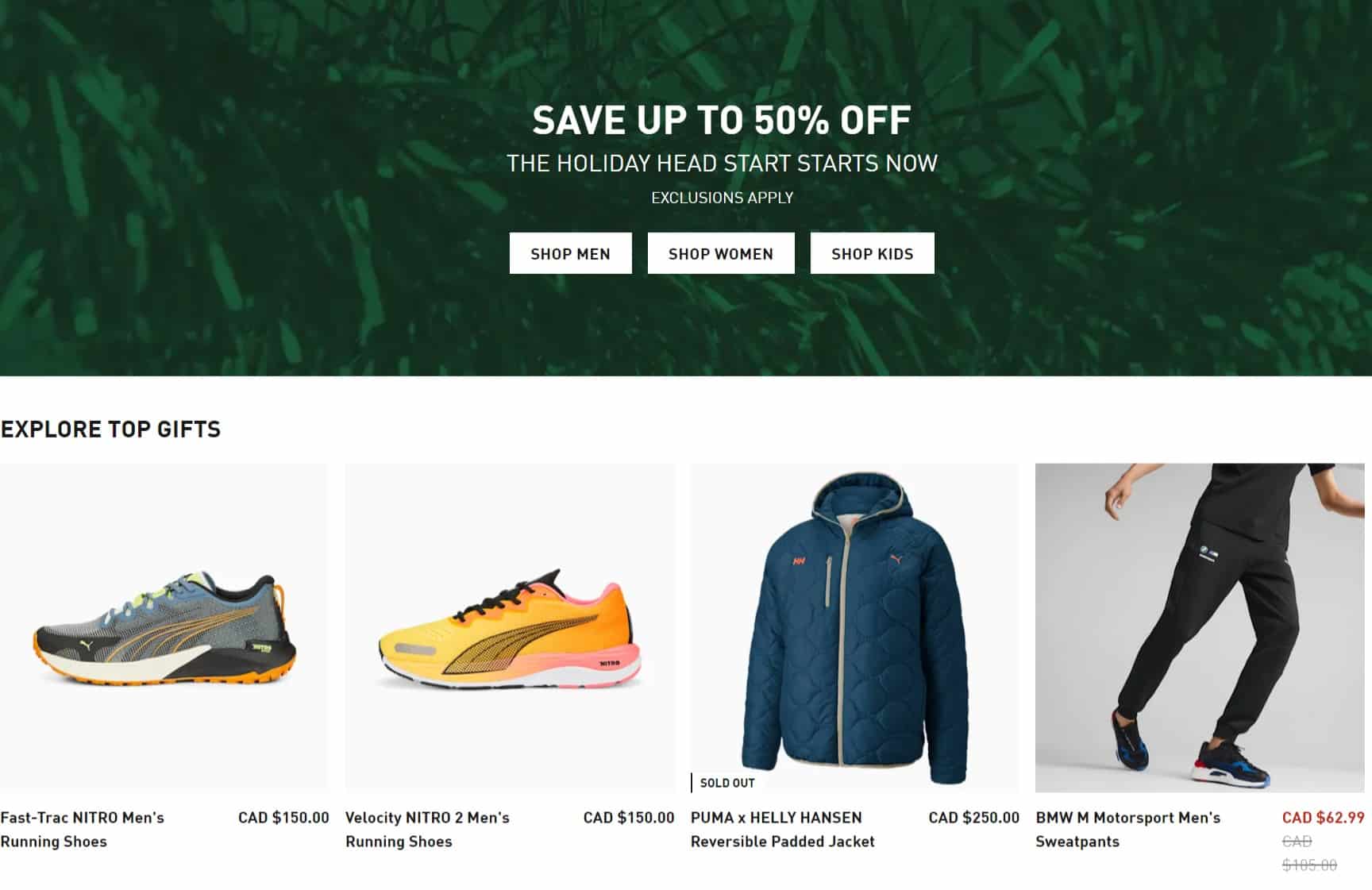This is a cropped screenshot from an activewear or sports and outdoor website. The top portion features a photo background with a close-up of Christmas tree branches, filtered in dark green. Overlaying this festive image in bold white text, it reads, "SAVE UP TO 50% OFF." Directly below, in smaller all-caps white letters, the text states, "THE HOLIDAY HEAD START STARTS NOW." Beneath this, in very small white text, it mentions "Exclusions apply." Centered underneath are three white boxes offering shopping categories: "SHOP MEN," "SHOP WOMEN," and "SHOP KIDS."

The section below the photo background is predominantly white. In the top left corner, it says "EXPLORE TOP GIFTS" in all-caps black letters. Below this heading is a horizontal row of product thumbnails. Each thumbnail includes the product's title and price. The first thumbnail showcases a side view of a shoe, labeled "Fast Track Nitro Men's Running Shoes" at the bottom left, with its price listed as "CAD $150" at the bottom right.